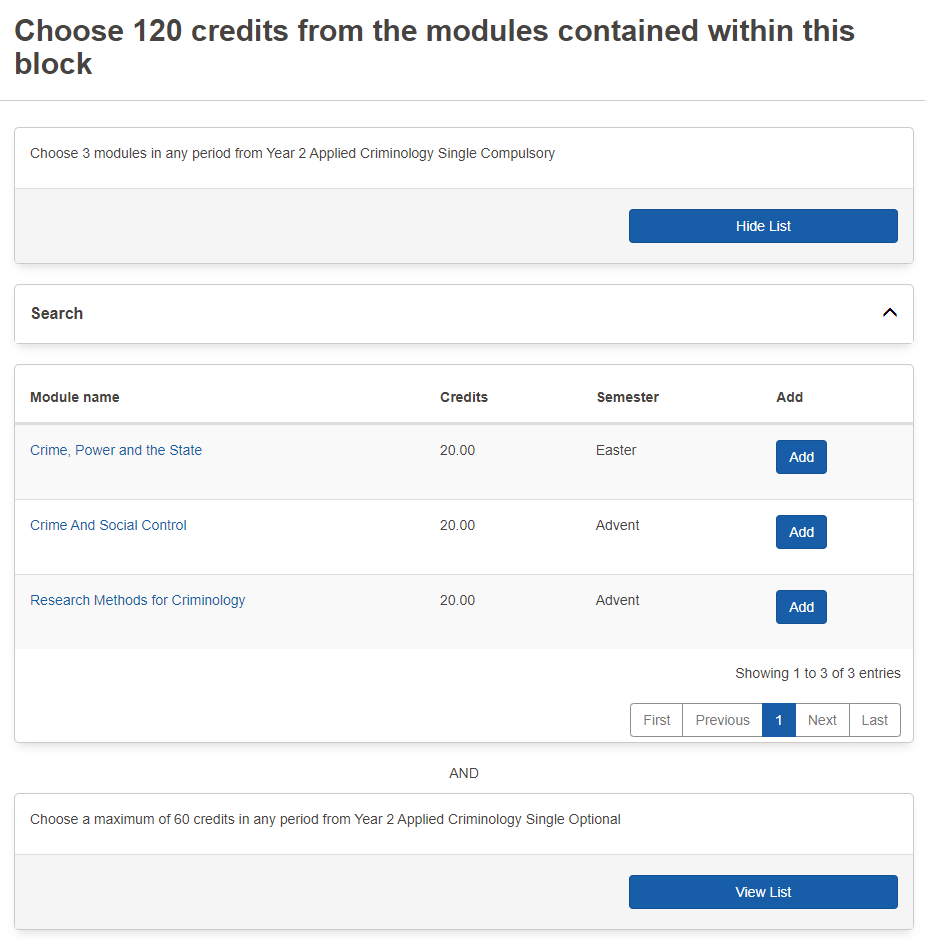This screenshot displays a detailed view of a web page, featuring several outlined sections with educational information. The background is white, and there are four main rectangular sections, each with a thin gray outline and slightly rounded corners.

At the very top is a multi-part section. It contains a white bar labeled "Choose three modules in any period from Year Two Applied Criminology, Single Compulsory" and a light gray bar beneath it. In the bottom right of the gray bar, there is a blue button with the white text "Hide List."

Below this is a single white row that functions as a search bar. It is labeled "Search," and an arrow pointing upward is located on the far right side of this row.

The largest section under the search bar features a table with alternating white and gray rows. The top row is white and lists the column headers: "Module Name," "Credits," "Semester," and "Add." Below these headers are three rows containing module details, each containing a blue title link, a credit value, a semester name, and an "Add" button in blue with white text for each module. The modules listed are:
1. "Crime, Power, and the State" - 20.00 credits, Semester: Easter
2. "Crime and Social Control" - 20.00 credits, Semester: Advent
3. "Research Methods for Criminology" - 20.00 credits, Semester: Advent

The final section communicates additional instructions, stating "Choose a maximum of 60 credits in any period from Year Two Applied Criminology, Single Optional."